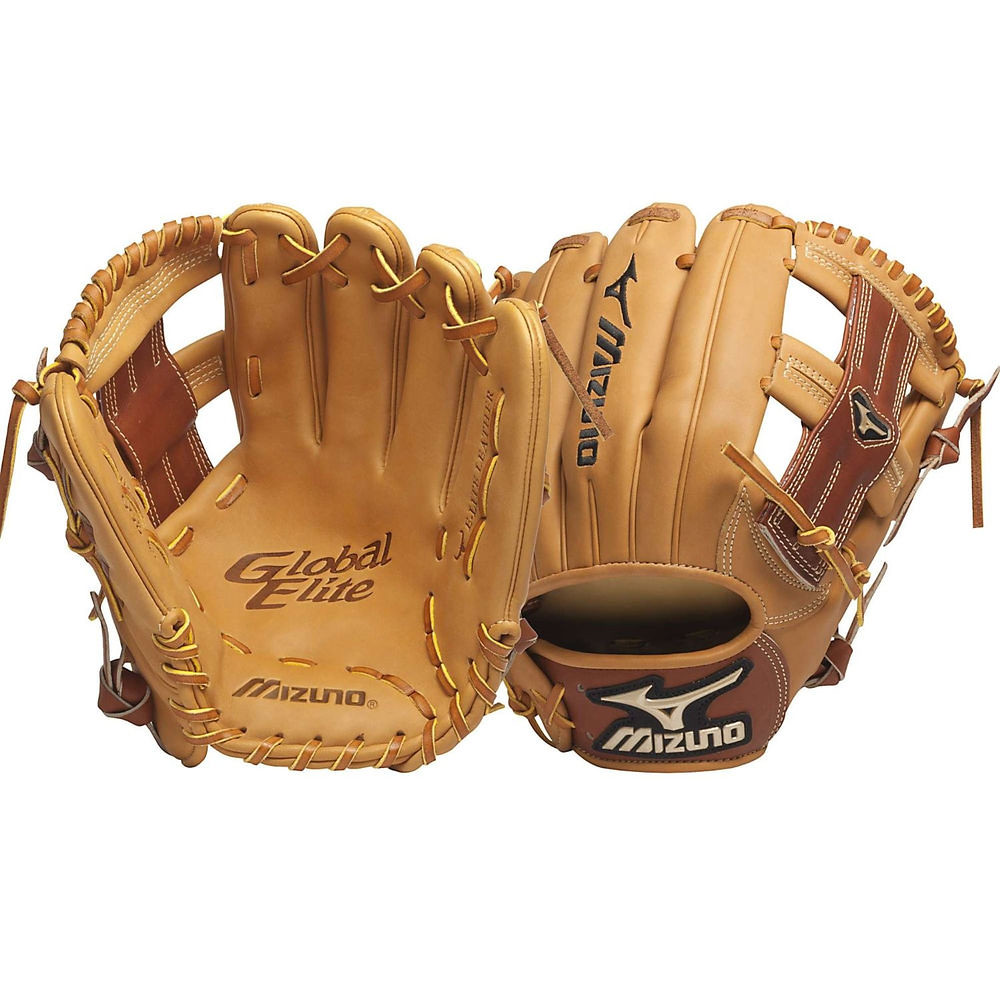This image depicts two pristine leather baseball gloves, side-by-side, showcasing different angles of the same model. Both gloves are crafted from a warm, creamy beige leather with hints of brown, exuding a luxurious feel. The glove on the left is presented palm-up, revealing intricate details like "Global Elite" emblazoned on the palm, "Mizuno"—spelled M-I-Z-U-N-O—in white text near the edge, and a variety of cross-hatched lacing patterns reinforcing the thumb, middle, and little finger areas. The darker brown stripe along the pocket is triple-stitched and houses a subtle emblem on the crossbar.

The glove on the right is viewed from the back, where "Mizuno" in black embroidery stands prominently below a white Japanese character symbol. This side also features the same dark brown stripe running down the area where the ball is caught, complementing the chocolate brown base color. The back label of this glove similarly notes "Global Elite," engraved in a lighter shade of brown. Overall, these impeccable and unworn gloves highlight the meticulous design typical of Mizuno's renowned craftsmanship.